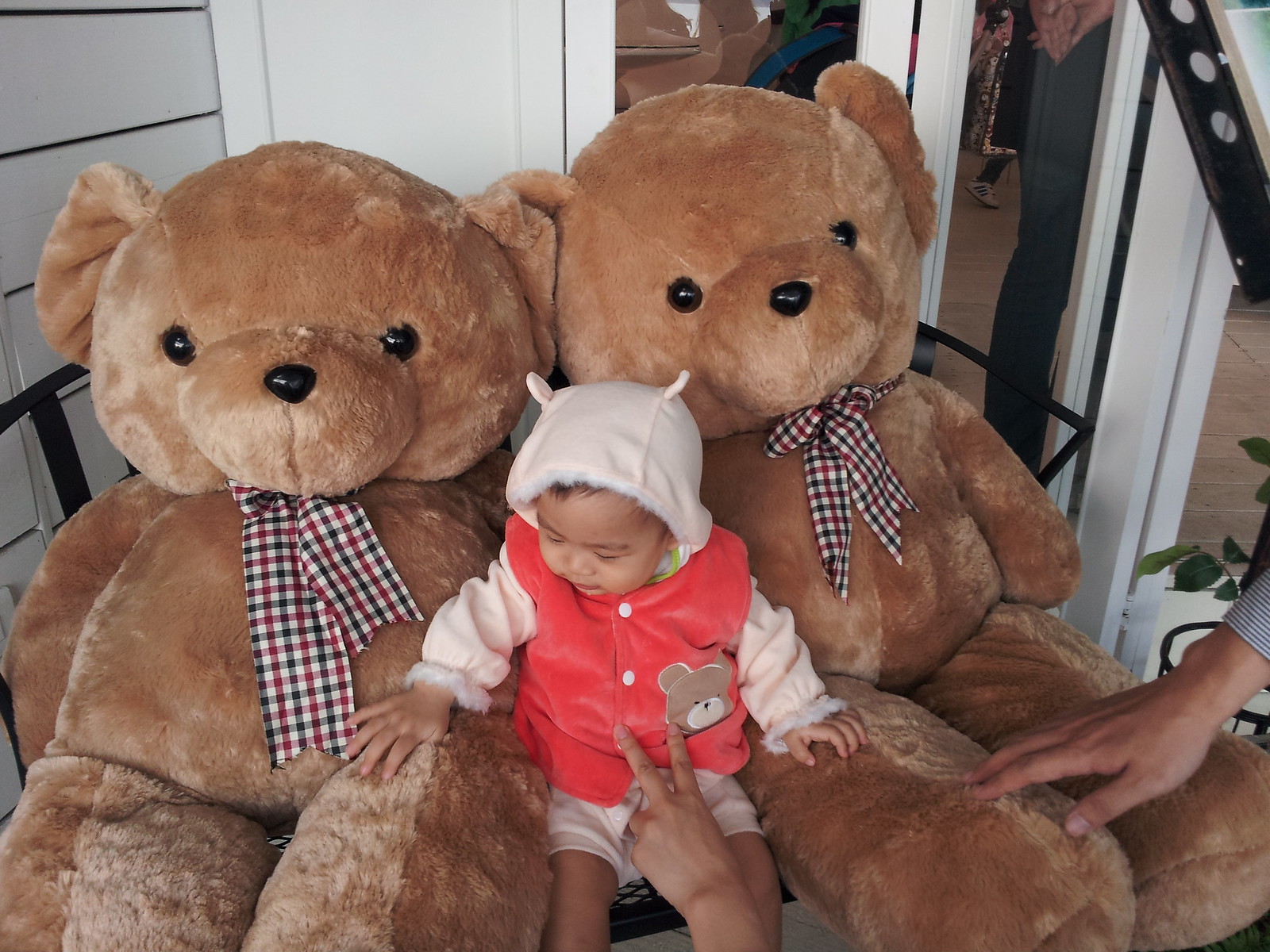In this heartwarming real-life photograph, we see a small Asian toddler nestled between two oversized, identical teddy bears. Each bear, a soft tan brown, features large black eyes, a plastic black nose, and a bowtie beneath its chin adorned with black, white, and red plaid ribbons. The toddler, dressed in an adorable outfit consisting of a red sweater with white sleeves, a pinkish cream hood with bear-like ears, and ivory shorts, grips the legs of the teddy bears with their tiny hands. The child is looking downwards to the left, adding an element of innocence to the scene. A left hand from off-camera is making a peace sign and gently poking the child’s belly, trying to capture the child's attention. Another hand with a striped sleeve reaches from the right, partially visible near one of the bears. The setting appears to be the exterior of a house, with a glass window and white and gray walls framing the background. A black bench that the trio sits on is barely visible at the edges of the photo. Overall, the image captures a charming moment with the toddler surrounded by the comforting presence of two giant teddy bears.